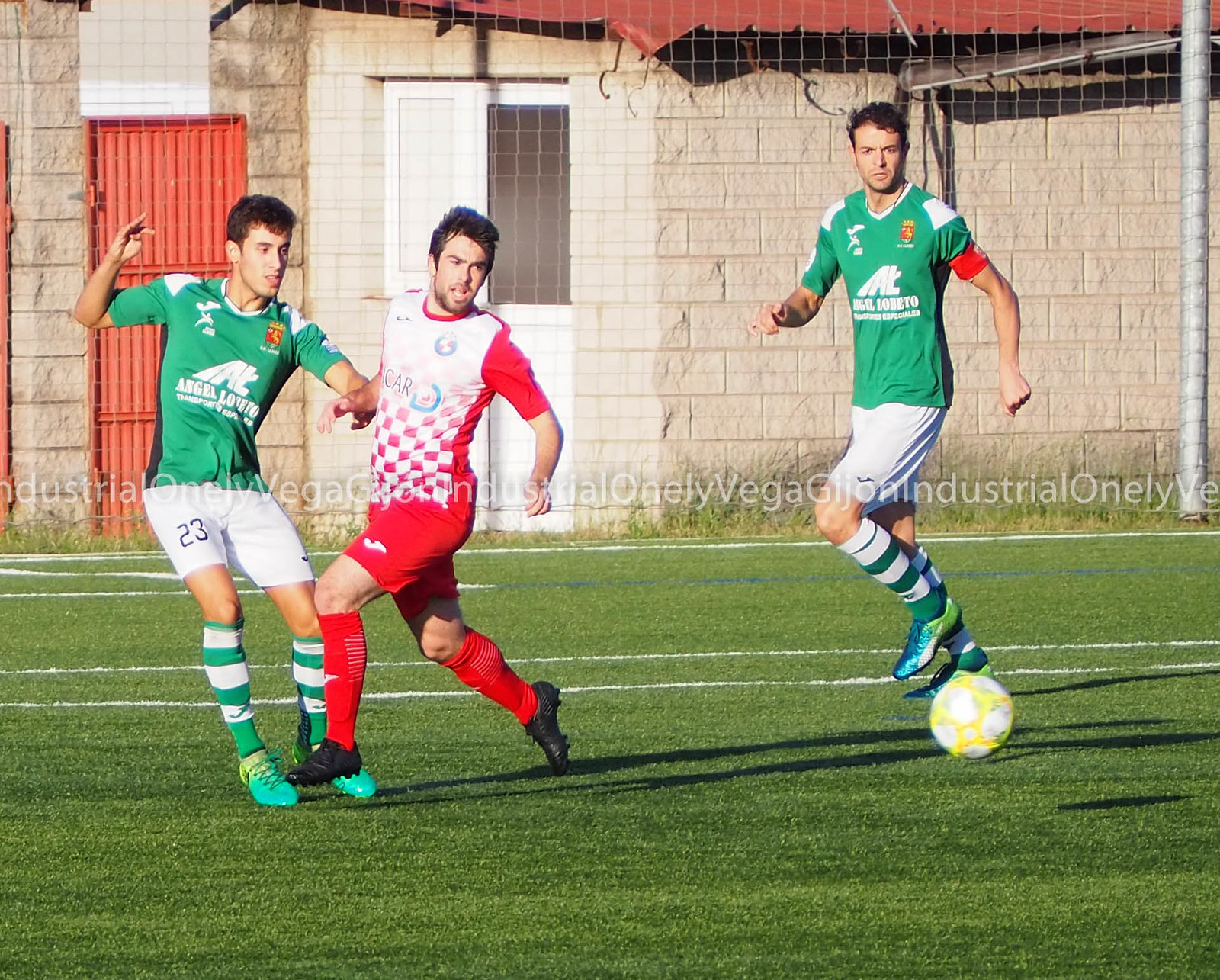In this outdoor action image, three men are intensely engaged in a soccer match on a lush green pitch. At the forefront, two players from the same team wear matching kits: green shirts adorned with white logos and lettering, white shorts, green and white striped socks, and green shoes. Both have short brown hair and are either white or Hispanic. One of these teammates, distinguished by a red armband on his left arm, stands slightly to the right and has his gaze firmly fixed on a white and yellow soccer ball. They are joined by an opponent positioned between them, clad in a red and white checkered shirt with red sleeves, red shorts, red socks, and black shoes. All three players are in motion, their focus converging on the approaching ball.

The background reveals a cement brick building with doors and a protective iron fence, contributing to the urban setting of the match. The scene is complemented by a soccer goal netting visible just in front of the building, adding context to this vibrant depiction of a mid-game moment. The bright green grass of the soccer field is marked with white lines, grounding the players in the dynamic and competitive atmosphere.